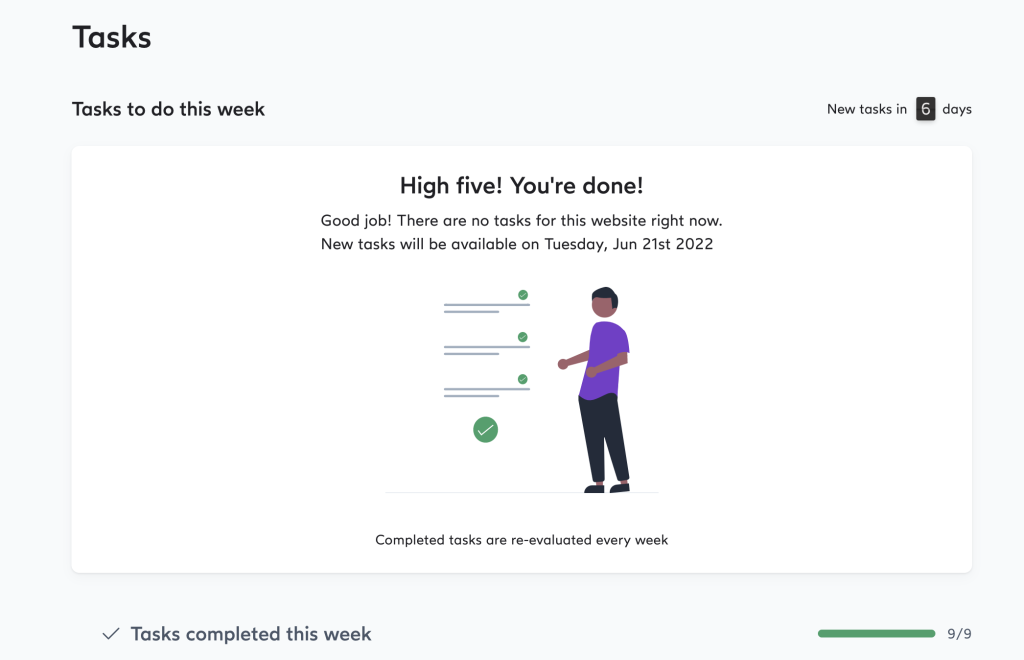Screen capture of a webpage showcasing task management and progress. In the upper left corner, the word "Tasks" is prominently displayed. Below this, a section titled "Tasks to do this week" is visible, indicating that there are no current tasks. The message "High five! You're done. Good job, there are no tasks for this website right now. New tasks will be available on Tuesday, June 21st, 2022." is displayed, accompanied by an icon of a person standing to the right of several bulleted points.

In the upper right corner, a notification reads "New tasks in 6 days," with the number six highlighted in a black rectangle with white font. On the lower left, the text "Tasks completed this week" is next to a green checkmark, signifying completion. The lower right corner of the screen features a progress line or bar, ending with "9/9" to indicate that nine out of nine tasks have been completed. To the left of this, a thick oval green horizontal line further emphasizes the completion status. The background of the webpage is white and devoid of other information, giving it a clean and focused look.